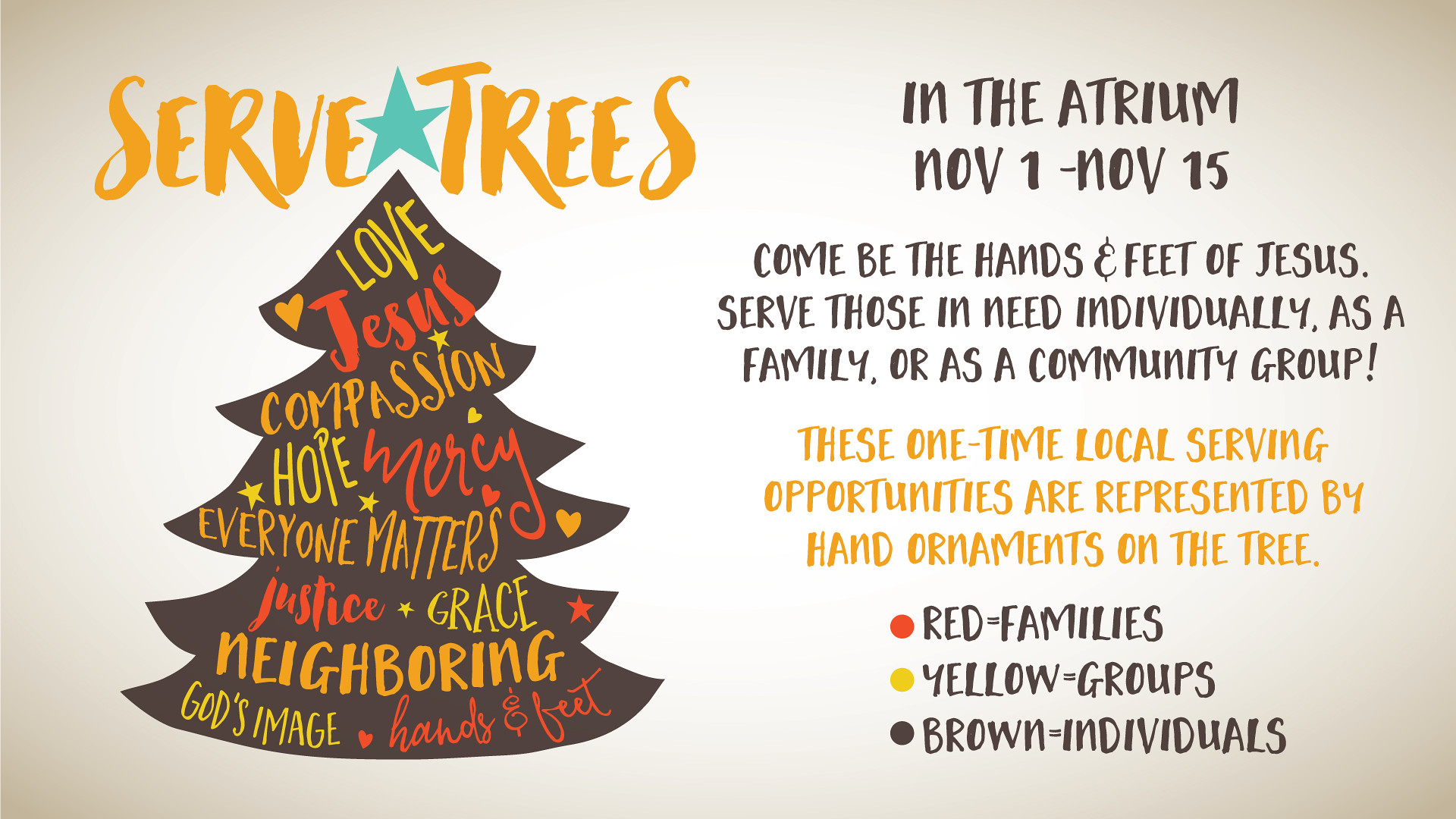The graphic advertisement, set against a white background with slight shadowing towards the corners, is oriented in a landscape manner. On the left half, the text "Serve Trees" is prominently displayed in yellow, accompanied by a blue star in the middle. Below this, an outline of a Christmas tree, shaded in dark brown, features a collage of words in yellow, orange, and red. These words include "Love," "Jesus," "Compassion," "Hope," "Mercy," "Everyone Matters," "Justice," "Grace," "Neighboring," "God's Image," "Hands and Feet," and various colored hearts and stars are interspersed among them.

On the right half, the text is divided into four sections. The first section, in brown text, announces, "In the Atrium, November 1 and November 15." The second section, also in brown, invites participation: "Come be the hands and feet of Jesus; serve those in need individually, as a family, or as a community group." The third section, in yellow text, clarifies, "These one-time local serving opportunities are represented by hand ornaments on the tree." Lastly, three bullet points in red, yellow, and brown circles respectively explain, "Red equals Families," "Yellow equals Groups," and "Brown equals Individuals." This detailed and visually engaging advertisement encourages communal service and participation in local charitable events.